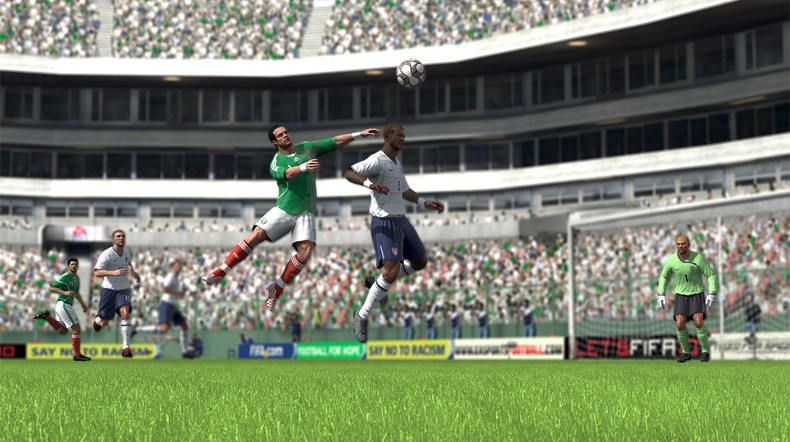This detailed scene appears to be a screenshot from a FIFA video game, likely from the 2010s era. The graphics, though not cutting-edge, are solid and 3D, depicting a packed stadium brimming with a live-action soccer match. The game captures an intense moment where multiple players from two distinct teams are in mid-action, vying for a black-and-white ball that's about three feet in the air. The teams are distinguished by their uniforms: one team wears green jerseys with white or silver shorts and red socks, suggesting they might be Mexico, while the other team wears white jerseys with blue or navy shorts, likely representing the United States. The field itself is a vivid green pitch, and we can spot the goalie off to the side. In the background, various advertisements are visible, including a notable “let's FIFA” banner and a "say no to racism" sign, reinforcing the game's FIFA branding. The scene is dynamic, with three characters sprinting up the field and two airborne characters, highlighting the game's realistic and engaging nature.